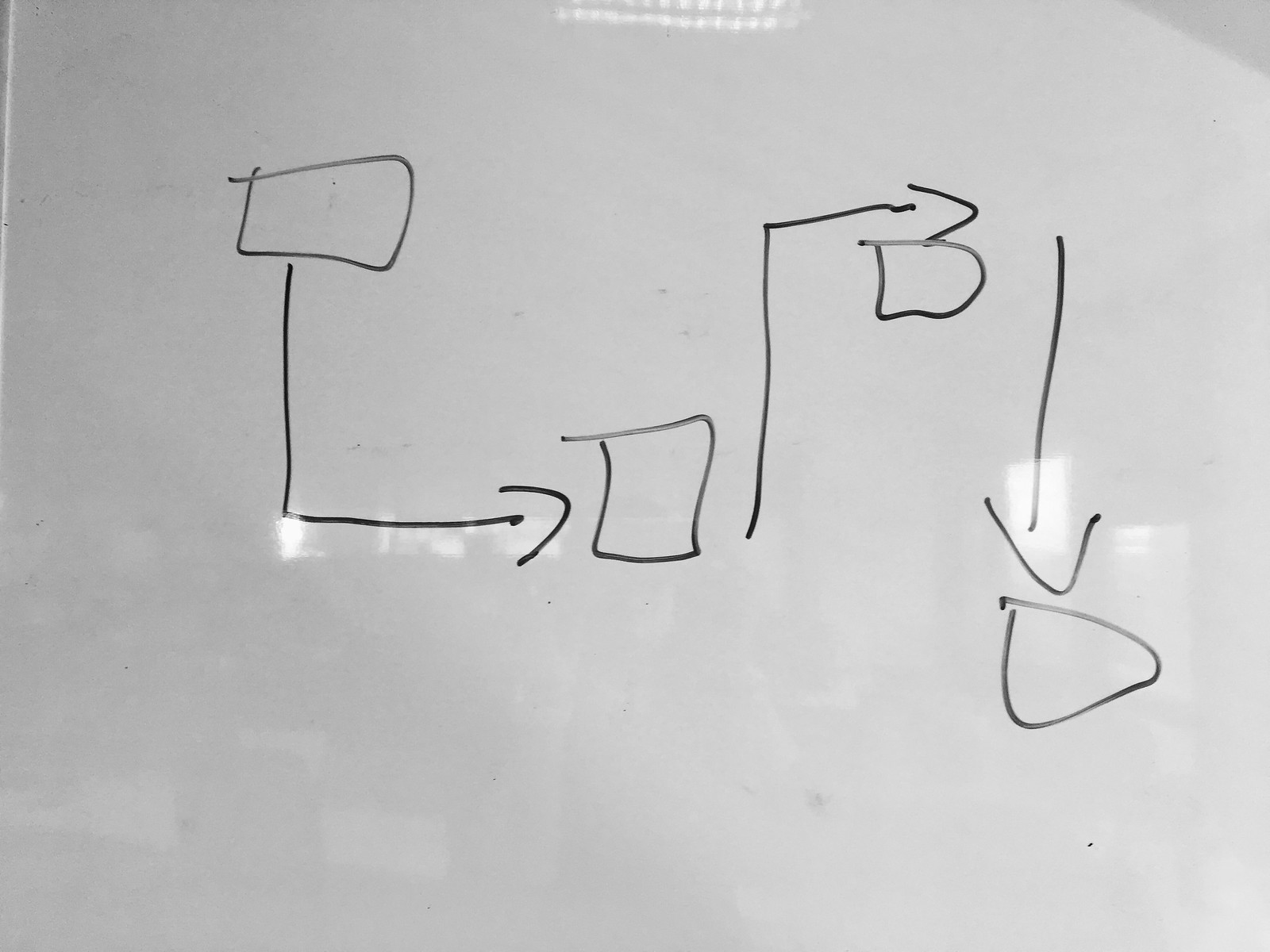A simple line drawing on a reflective, grayish-white surface, possibly plastic, features an array of crude geometric shapes and lines. At the top of the surface, indistinct white markings or numbers are faintly visible. The main composition begins with a roughly sketched rectangle in the upper left corner. Extending from its bottom is a vertical black line that bends into a horizontal line, forming a right angle, with an arrow pointing to the right. Adjacent to this arrow stands a small, upright rectangle. Further to the right, another vertical black line intersects with a horizontal line at a 90-degree angle, also ending in a right-pointing arrow, beneath which is the letter "G". Continuing downward, a vertical black line concludes with a downward arrow aimed at a poorly drawn triangle. The drawing's overall presentation is simplistic and rudimentary, with light reflections indicating that the surface may be plastic rather than paper.